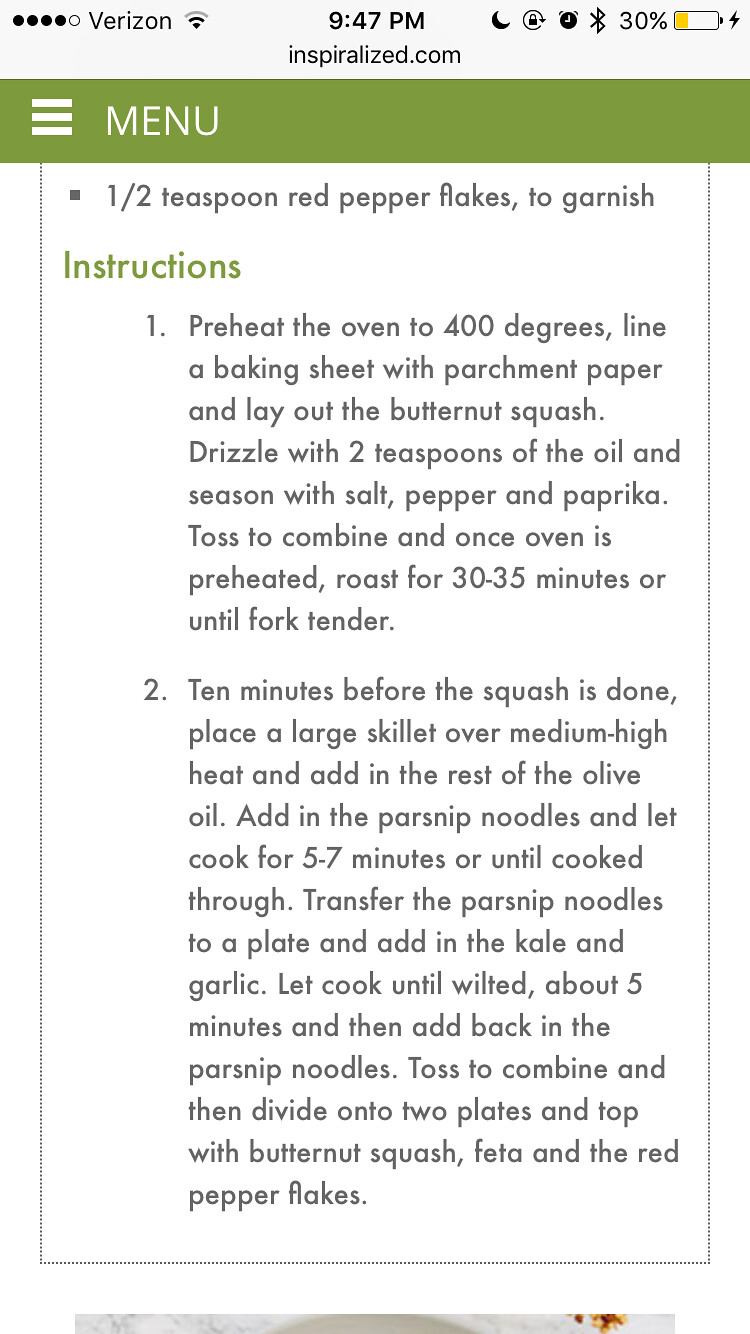This image is a screenshot of a mobile device displaying a recipe from the Inspiralized.com website. The screenshot captures a detailed cooking guide starting with preheating the oven to 400 degrees and preparing butternut squash with oil, salt, pepper, and paprika to roast for 30-35 minutes. Next, it describes sautéing parsnip noodles in olive oil and later cooking kale and garlic until wilted, combining these ingredients, and plating them with the roasted butternut squash and topped with feta cheese and red pepper flakes.

The recipe is displayed in a browser window, as indicated by the top green navigation bar labeled "menu," featuring a three-horizontal-lines icon typical of menu options. The device is connected to Verizon Wi-Fi, showing a battery level of 30% and a time of 9:47 p.m. The webpage itself predominantly uses a white background with black text for readability.